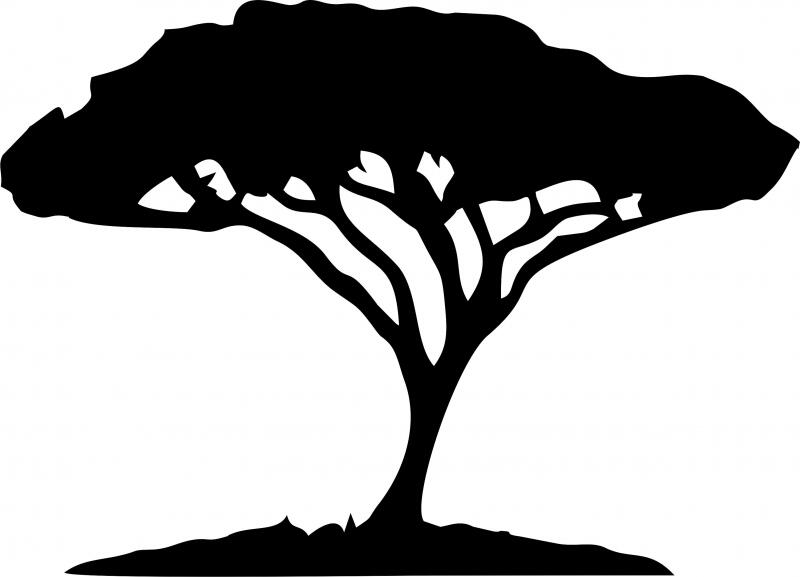The image depicts a stylized, simplistic silhouette of a tree against a white background. The tree features a small, slender trunk emerging from a black ground or dirt mound at the bottom. The bare, thin branches extend upwards and outwards, culminating in a dense, solid black canopy that suggests leaf cover. The silhouette resembles a cutout or template, akin to art inspired by African landscapes or possibly similar to certain Californian trees. The overall effect is minimalistic yet evocative, with the stark contrasts and clean lines making it ideal for artistic representations such as metal wall hangings.